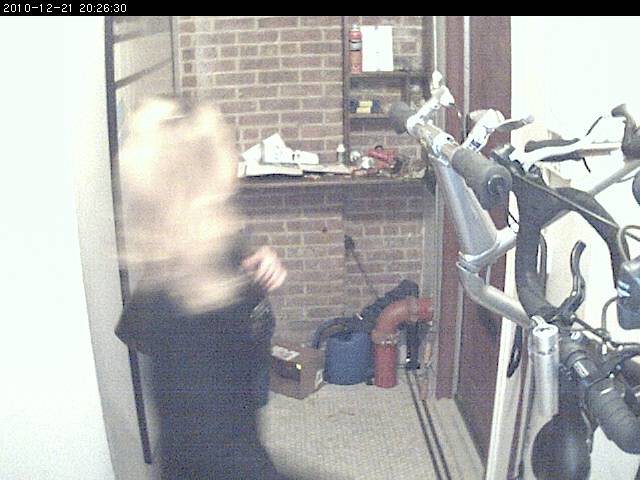The image depicts a cluttered room or supply closet, possibly within a residential or building maintenance setting. The focal point is a brick wall directly ahead, adorned with various tools and items. The wall is framed by two other walls, creating a corridor-like impression. A ledge or counter extends halfway up the brick wall, which is in disarray with multiple objects, including what appears to be a spray can of paint, a box, and a blue watering can. 

There is also machinery beneath the shelves near the brick wall, though it is difficult to discern due to the graininess of the photo. On the right side of the image, a dark brown or maroon door is visible, with something resembling bike handles or exercise equipment in front. A red pipe extends into the house from this right side. 

A woman with long blonde hair, dressed in an all-black outfit, is seen walking through the room on the left side. Her face is indistinct due to motion blur, suggesting she is shaking her head. The floor is covered with a beige carpet, adding to the domestic rather than industrial ambiance of the setting.